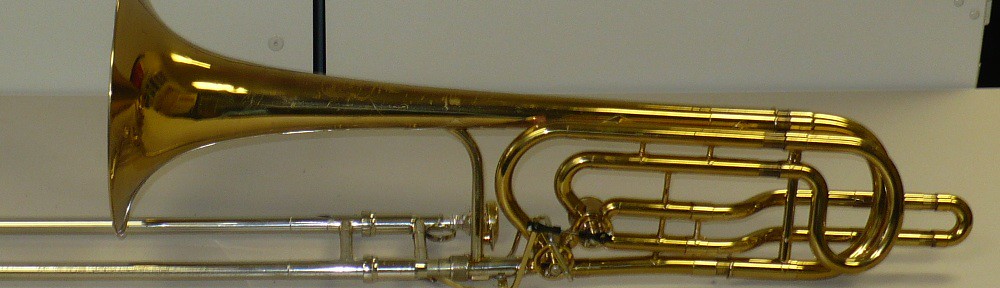The image features a detailed, horizontal view of a brass trombone, resting on its slide section. The trombone, predominantly golden in color with some parts appearing brass or bronze, displays a mix of shiny and worn areas. Notably, the slide shows signs of wear and is silvered from use. The instrument's intricate tubing can be seen curling around three times before flaring out into a glossy, reflective bell on the left side of the image. This reflective surface catches the room's lighting and possibly the photographer's reflection. The instrument, which includes a central mouthpiece shaped like a small bell, is placed against a white backdrop comprised of a wall and floor. Shadows from the trombone and the ambient lighting add depth to the scene. Additionally, there is a black bar visible on the left side near the horn flare, juxtaposed against the lighter background.